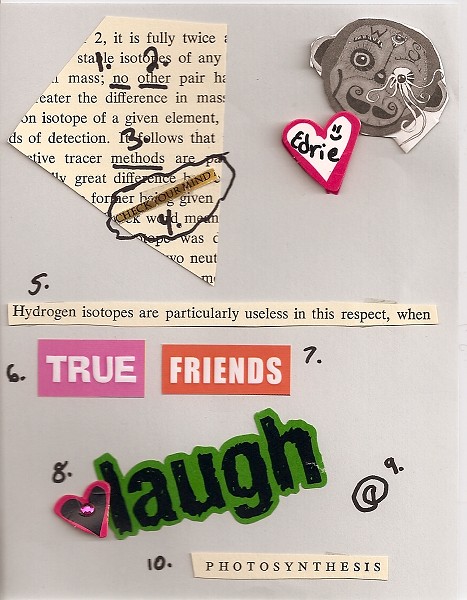The image is a detailed, handmade collage set against an off-white, grayish background. It comprises various cutouts from magazines and newspapers, meticulously numbered and annotated. Prominent elements include a newspaper clipping with the phrase "no other" underlined and marked with numbers 1 and 2, and the word "methods" underlined with a number 3. A section of the document is crossed out and covered with tape, labeled number 4. 

There’s also a magazine snippet with the text "hydrogen isotopes are particularly useless in this respect," marked number 5. Additionally, pieces of colored paper feature prominently: a blue paper with the word "true," an orange paper with "friends," all labeled 7, followed by a heart and the word "laugh," numbered 8, and an '@' symbol drawn in pen as number 9. The number 10 leads to the final word, "photosynthesis." 

The collage includes visual elements such as a monkey illustration and a heart, positioned at the top right of the image. The entire composition is marked by vibrant colors including red, pink, white, green, black, light red, beige, and gray. This creative and meticulously arranged collage likely results from manual assembly or digital work, possessing elements suggestive of a mixed media or Photoshop project.